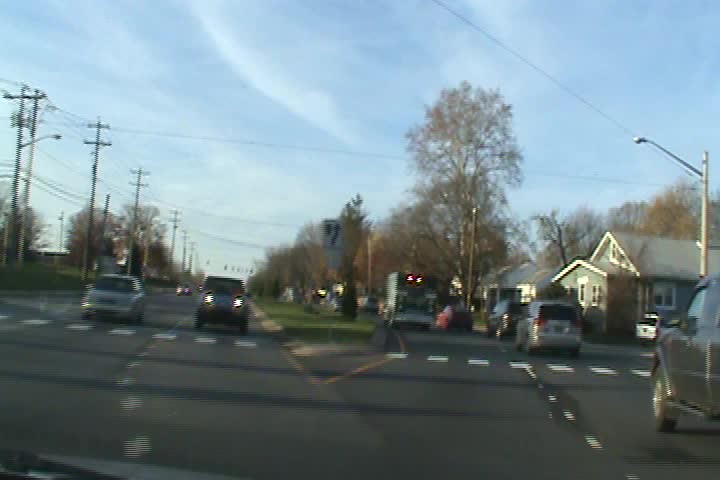The image depicts a two-way road with two lanes on each side, separated by a grassy median. On the left side of the road (cars heading south), there's a sequence of vehicles including a gray minivan, a black car, and a red car. On the right side (cars heading north), several cars are visible, such as a black pickup truck and a gray sedan with its lights on. A white pole with black signs is standing in the median, and power lines cross overhead.

To the right of the road, there's a residential area with houses, including a notable green house with a black roof and a white house. The background features additional dwellings and trees that appear mostly barren with few leaves. The road in front of the green house has white dashed markings. A bus is seen driving in the opposite lane. The sky above is blue with a few clouds scattered throughout.